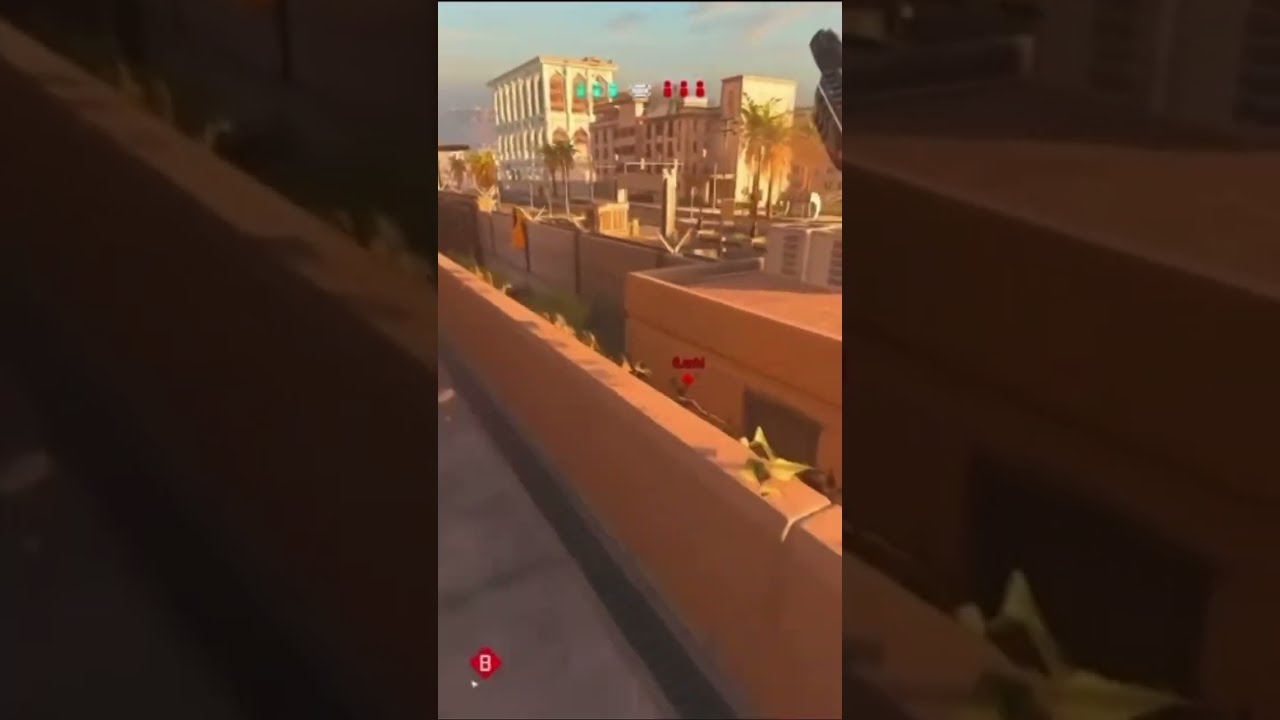This photograph, likely a cell phone portrait-style image adapted into a landscape format with faded black edges on either side, captures a bustling construction zone on a city street. In the foreground, a vivid orange plastic barrier stands out, indicative of ongoing roadwork. Beyond the barrier, construction equipment and cement structures are visible, contributing to the scene's industrious atmosphere. The midground and background display several notable elements, including an ornate two-story building with white walls and multiple columns, visible against a backdrop of lush palm trees, suggesting a warm, possibly Californian setting.

Some aspects hint at a rooftop perspective, with adjacent rooftops and an air conditioning unit visible, while the sandy red-orange hues of a surrounding wall add a distinct character to the scene. The photo was taken during the daytime, underlining the ambient light and vibrant colors – shades of brown, dark and light orange, yellow, black, red, teal, tan, and beige, alongside the verdant greenery. The palm trees, prominently featured and centered in the composition, along with the white buildings, serve as focal points, drawing the viewer’s attention to the urban skyline stretching into the distance.